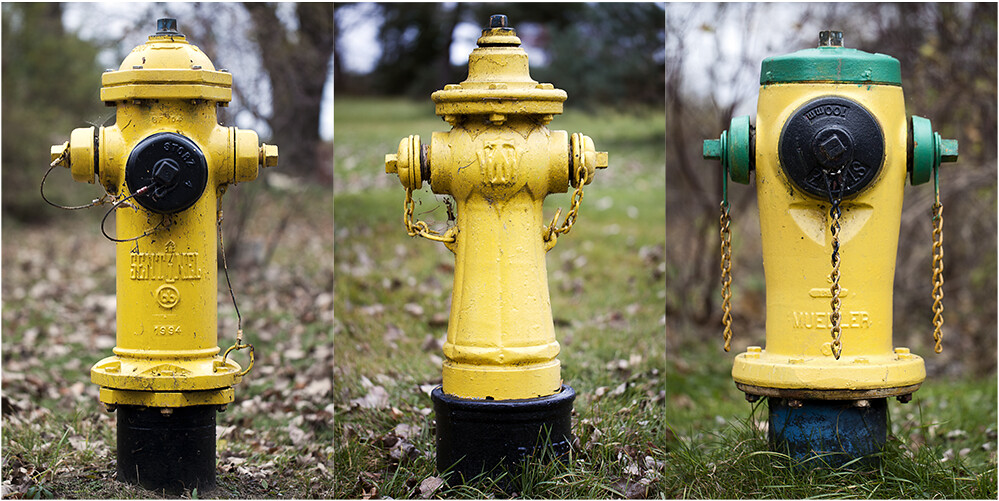This photograph features three yellow fire hydrants, each depicted in separate yet side-by-side sections. The hydrants are set against a natural, slightly blurry backdrop of grass, leaves, and trees.

The hydrant on the left has a distinctive black base and a prominent black circle on its front, likely where a hose would be attached. Its metal body, painted in a bright yellow hue, contrasts with the natural surroundings of brown leaves and green foliage.

The central hydrant shares a similar yellow and black color scheme, with a slender, bell-shaped design. Unlike the first, this hydrant lacks the black circle on its front and features a yellow chain draped around it, blending into the green grass and brown leaves of the background.

The hydrant on the right stands out with its unique accents. It has a yellow body that narrows at the base and is crowned with a green top. This hydrant is equipped with green fittings on the sides, from which chains dangle. A black circle adorns its front, similar to the one in the leftmost image. The surrounding scene maintains the theme of grass, leaves, and trees, with a slight blur to the background.

Overall, the image captures three distinct yet uniformly yellow fire hydrants, each with subtle variations in design and embellishment.